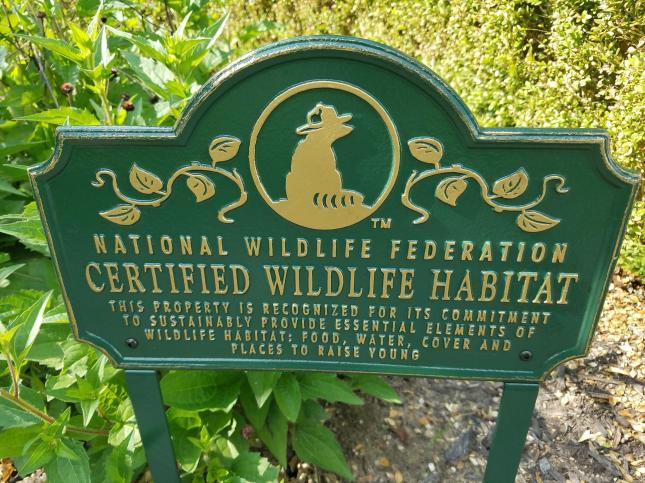This detailed close-up outdoor photo depicts a sign from the National Wildlife Federation, or NWF, that acknowledges a Certified Wildlife Habitat. The green, metal placard, mounted on two metal posts, features gold lettering which reads: "National Wildlife Federation Certified Wildlife Habitat. This property is recognized for its commitment to sustainably provide essential elements of wildlife habitat, food, water, cover, and places to raise young." The sign's design includes an oval top and a rectangular bottom, adorned with stylized vines and leaves. At the top of the sign is an emblematic icon that resembles a racoon, or perhaps a bear, donning a park ranger hat. Two black nails are visible in the bottom corners of the sign. The background reveals shrubbery and various plants with differing leaf sizes, indicating it's a sunny day. The angle of the photograph is directed downwards toward the ground, with no sky visible.